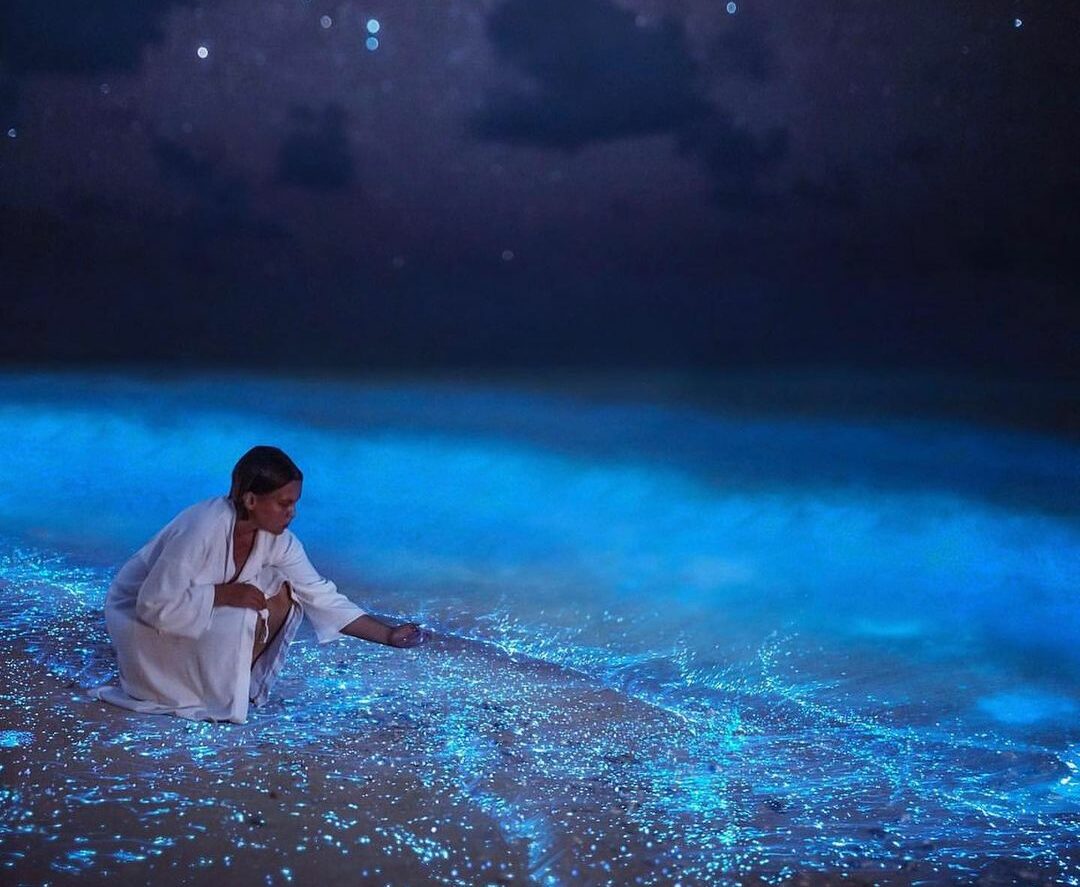The image is a detailed, color photograph in landscape orientation, capturing a serene, starry night at a beach. In the foreground, a woman with dark skin and short, dark brown hair, held back and appearing wet, is crouching down on the left side. She is dressed in a long-sleeved white robe and reaching out to touch the luminous, bioluminescent water. The water exhibits a striking blue neon glow, potentially enhanced through Photoshop, with fluorescent splashes casting an ethereal light onto the tan sand beneath her. The background features a captivating night sky transitioning from light blue to deep purple and finally to black closer to the horizon, peppered with dark gray clouds and numerous luminous stars. This scene depicts the mesmerizing "sea of stars" on Vadu Island in the Maldives, blending photographic representationalism and realism to create a dreamlike, visually enchanting moment.